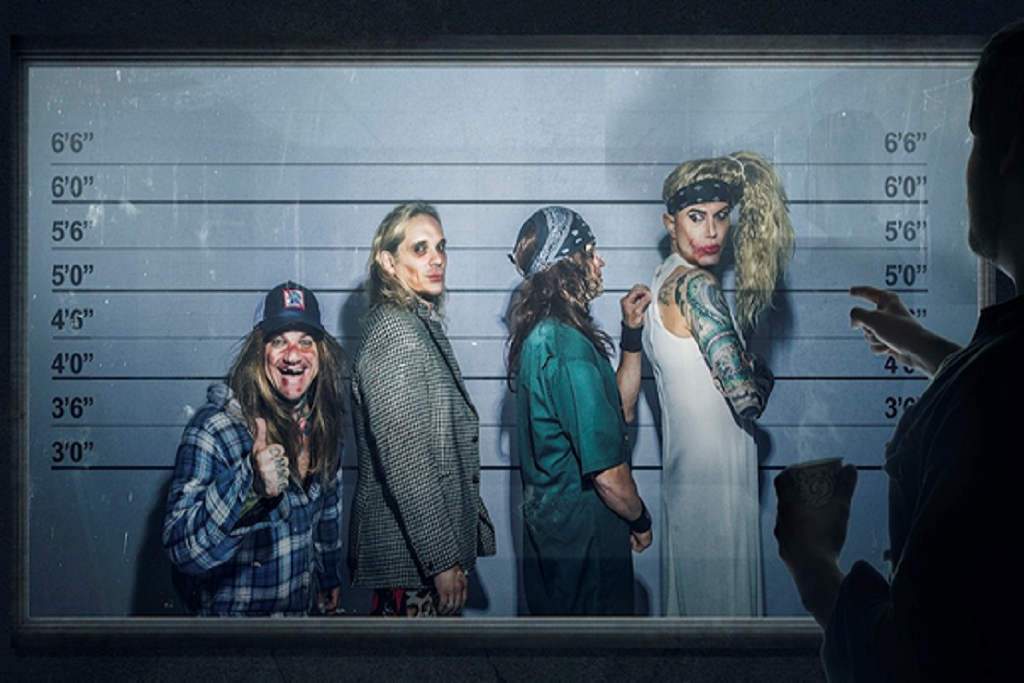In this intriguing image of a police lineup, a person silhouetted in a dark room is observing and pointing at four unconventional-looking individuals through a large window. The dark room features the individual's shadow and silhouette, highlighting their focused stance. The window opens to a brightly lit area where the lineup stands in front of a white board marked with height measurements, clearly delineating each person’s stature. 

From left to right, the first individual, approximately five feet tall, sports a trucker hat, a blue plaid shirt, and is covered in blood. They have long hair and a beaming smile, giving a thumbs-up to the observer. The second in line, roughly six feet tall, dons a checkered tweed jacket, has a gaunt face, long scraggly hair, and an intense gaze, facing sideways but with their head turned towards the camera. 

The third person, also around six feet, wears a blue bandana, black wristbands, a long green t-shirt, and has long messy hair. They are touching the back of the tallest individual, who stands at about six foot six. This person wears a striking white long sleeveless gown, flaunts a sleeve of tattoos, and has a heavily made-up face with red lipstick. Their blonde hair is tied up in a voluminous bushy ponytail to the side, and they are looking back at the person touching them. Each person in this lineup, distinguished by their unique attire and appearance, adds to the peculiar atmosphere of the scene.